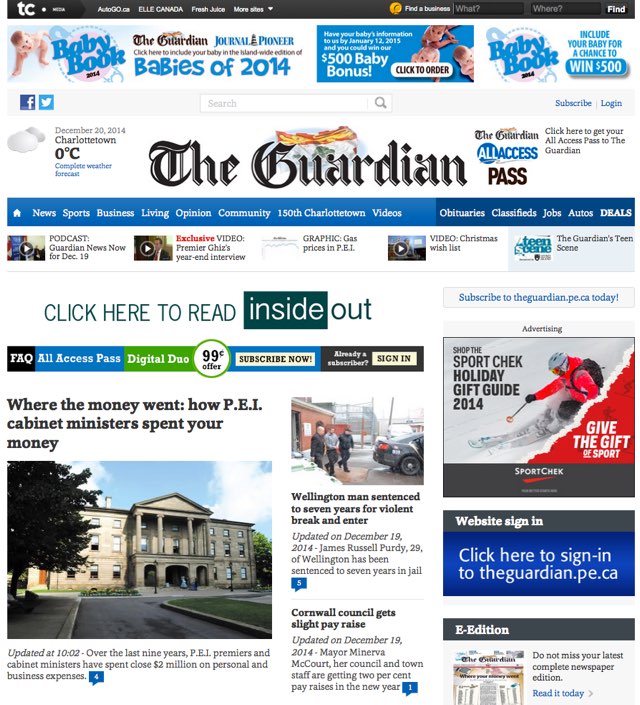This image is a screenshot from a website or app, characterized by a comprehensive and detailed layout. At the top of the interface is a prominent black bar spanning the width of the screen. In the left-hand corner, "TC" is displayed in white text, followed by a list of websites including "autogo.ca," "lcanadafreshjuice," and an option labeled "More Sites," indicated by a downward arrow for a dropdown menu. Moving towards the right, the bar features a search area labeled "Find a Business," accompanied by two text boxes for inputting search parameters labeled "What" and "Where." A button labeled "Find" is situated on the far right.

Below this bar is an advertising banner promoting the "Baby Book 2014" by The Guardian Journal Pioneer, inviting users to include their baby in the island-wide edition of "Babies of 2014." The ad indicates that submissions should be made by January 12, 2015, for a chance to win a $500 baby bonus, emphasizing the call-to-action with multiple "Click to order" prompts.

Further down, the website is identified as "The Guardian." On the left-hand side, the current weather is displayed, showing the date as December 20, 2014, and weather information for Charlottetown at 0 degrees Celsius, with a link to a "Complete Weather Forecast." Directly beneath this section is a navigation bar listing various sections: News, Sports, Business, Living, Opinion, Community, 150th Charlottetown, Videos, Obituaries, Classifieds, Jobs, Autos, and Deals. The main feature article headline reads "Where the Money Went: How PEI Cabinet Ministers Spent Your Money," hinting at a detailed investigative piece on government expenditures. The overall layout underscores a structured and user-friendly design aimed at providing comprehensive information and easy navigation.